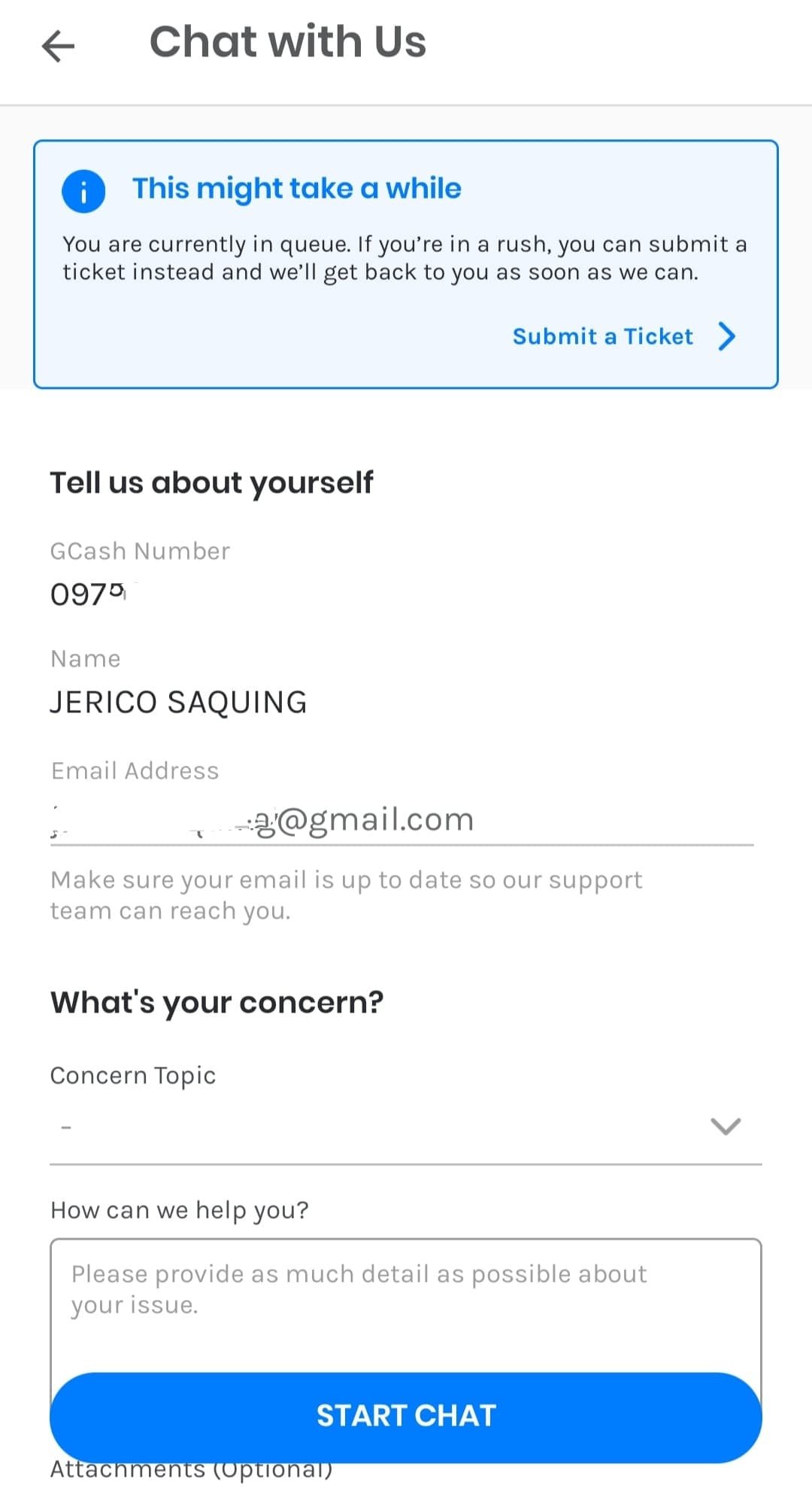**Image Description:**

The image depicts a tall, vertically-oriented chat interface, reminiscent of smartphone displays but devoid of typical Android or iPhone icons.

At the very top, within a white header, a black leftward-facing arrow is situated, followed by the text "Chat with us" in black.

Below this header is a gray square containing a blue-rimmed rectangle with a light blue interior. Inside the rectangle, a blue circle with a lowercase letter "i" is centered. To the right of the circle, blue text states, "This may take a while." Beneath this message, in black letters, it reads, "You are currently in queue. If you're in a rush, you can submit a ticket instead, and we'll get back to you as soon as we can." To the lower right within the rectangle, "Submit a ticket" is written in blue, followed by a rightward-facing chevron.

Further down, a large white section begins with "Tell us about yourself" in black text on the left side. Below that, in gray letters, "GC cash" is displayed, followed by the number "097." A small zero, resembling a degree symbol, appears above and to the right of the seven. 

Following this, the word "Name" is printed in gray, succeeded by the name "Jericho Saquing" in all caps, using black letters. Further down, "Email address" is indicated in gray text, with a thin gray line beneath. Above the line, partially legible and difficult to read, appears a "G" followed by "@gmail.com."

Underneath this, a note in gray advises, "Make sure your email is up-to-date so our support team can reach you." Next, in black letters, "What's your concern" is posed, leading to a labeled section "Concern Topic" with an accompanying dropdown menu marked by a downward-facing gray chevron and a gray bar below it.

Lastly, black text on the left asks, "How can we help you?" adjacent to a gray-rimmed text box, partially obscured towards the bottom. Within the box, the prompt, "Please provide as much detail as possible about your issue," is displayed in gray. Concealing the bottom bar of this box, a long blue oval button stands out, inscribed with "START CHAT" in white, all-capital letters. To the lower left, "Attachments (optional)" is noted in black text with parentheses.